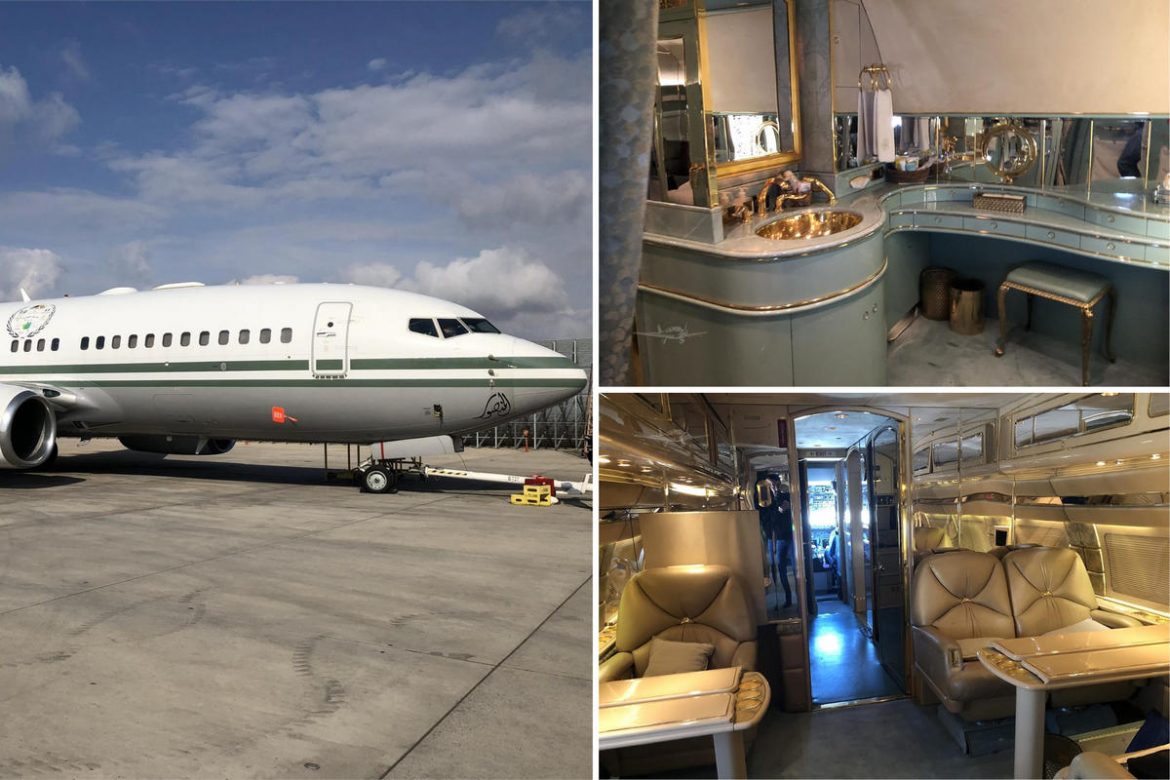This composite image consists of three separate photographs, each offering a different perspective of a luxurious airplane. The first photo on the left shows the exterior of the aircraft. It captures the upper part of a white airplane adorned with dark green stripes running horizontally from nose to tail. The plane is stationed on the ground with its wheels visible and fully extended. The aircraft's engines are prominently mounted on the sides, indicating it's ready for takeoff. The sky above is partly cloudy, providing a serene backdrop. Although the image cuts off part of the airplane, it suggests a smaller, private jet, recognizable by the array of small windows lining its side.

The other two pictures reveal the opulent interior of the plane. One of these images showcases a lavishly designed bathroom featuring gold accents throughout, including a sink that shines with a gold-like surface. The bathroom appears to have a dedicated makeup area, equipped with multiple mirrors, enhancing its luxurious ambiance.

The third photo gives a glimpse into the plane's seating area, which is equally indulgent. The seats are upholstered in a combination of white and green fabrics, exuding comfort and elegance. Each detail underscores the plane's sophisticated and high-end design, making it clear that this aircraft is outfitted for a luxury travel experience.